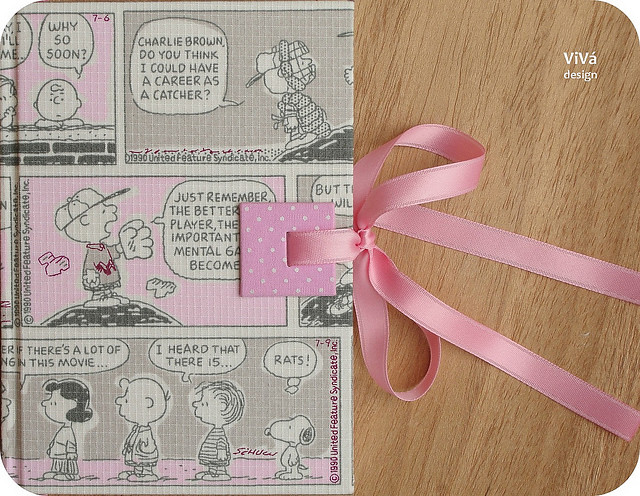The photograph captures a Charlie Brown themed journal styled as a comic strip, lying on a light wooden table. The cover features prominent comic elements, including a dialogue that reads, "Charlie Brown, do you think I could have a career as a catcher?" The design showcases a mix of colors such as black, white, gray, and pink. Notably, a pink ribbon with white polka dots is tied in a bow on the right side, serving as the binding closure for the journal. The overall composition places the journal on the left half of the image, with the ribbon extending diagonally to the right. In the top right corner of the cover, there's a logo that says "Viva Design." The setting appears to be indoors against a wooden backdrop.